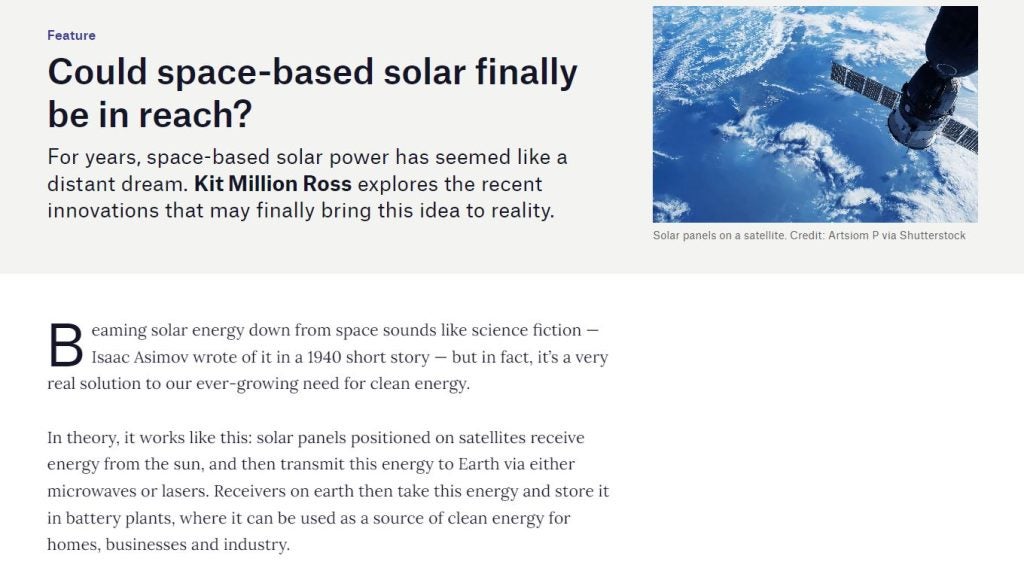Screenshot of a webpage discussing the advancements in space-based solar power. At the top, a gray horizontal banner spans across the page, featuring a square photograph of solar panels on a satellite, credited to Artsiam P via Shutterstock. The satellite is captured over a backdrop of blue water and scattered clouds, positioned in the upper right corner and facing towards the cloud-filled expanse below. The main text of the article reads: "Could space-based solar finally be within reach? For years, space-based solar power has seemed like a distant dream. Kit Million Ross explores the recent innovations that may finally bring this idea to reality. Beaming solar energy down from space sounds like science fiction. Isaac Asimov wrote of it in a 1940 short story, but in fact, it's a very real solution to our ever-growing need for clean energy. In theory, it works like this: Solar panels positioned on satellites receive energy from the sun and then transmit this energy to Earth via either microwaves or lasers. Receivers on Earth then take this energy and store it in battery plants, where it can be used as a source of clean energy for homes, businesses, and industry."